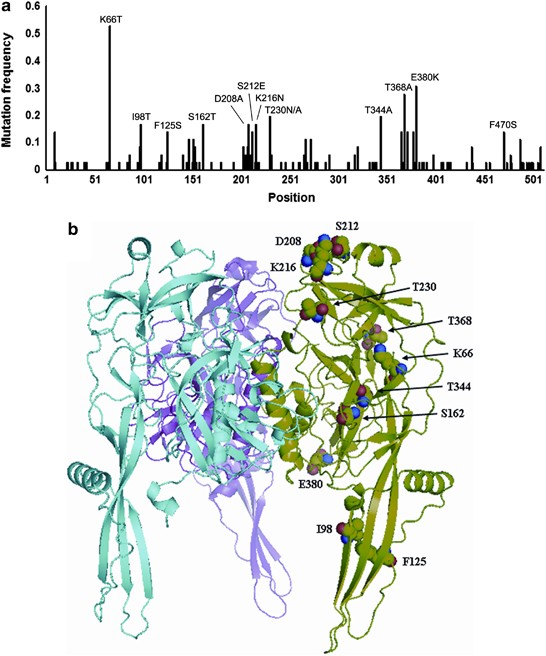The image displays a detailed scientific diagram divided into two primary sections. The top section features a bar graph labeled "Mutation Frequency" with the x-axis marked as "Position." The graph illustrates varying mutation frequencies across different positions, corresponding to a set of four-digit numbers. Below the graph, occupying most of the visual space, is a vibrant and intricate depiction resembling confetti or flowing ribbons in shades of teal, purple, green, and a touch of brown. These multicolored ribbons, which overlap in certain areas, also contain scattered four-digit numbers correlating with the graph above. The overall layout of the image is dynamic, aiming to visually connect the positions indicated on the bar graph with the colored ribbons below, likely representing mutation occurrences in a visually engaging manner.